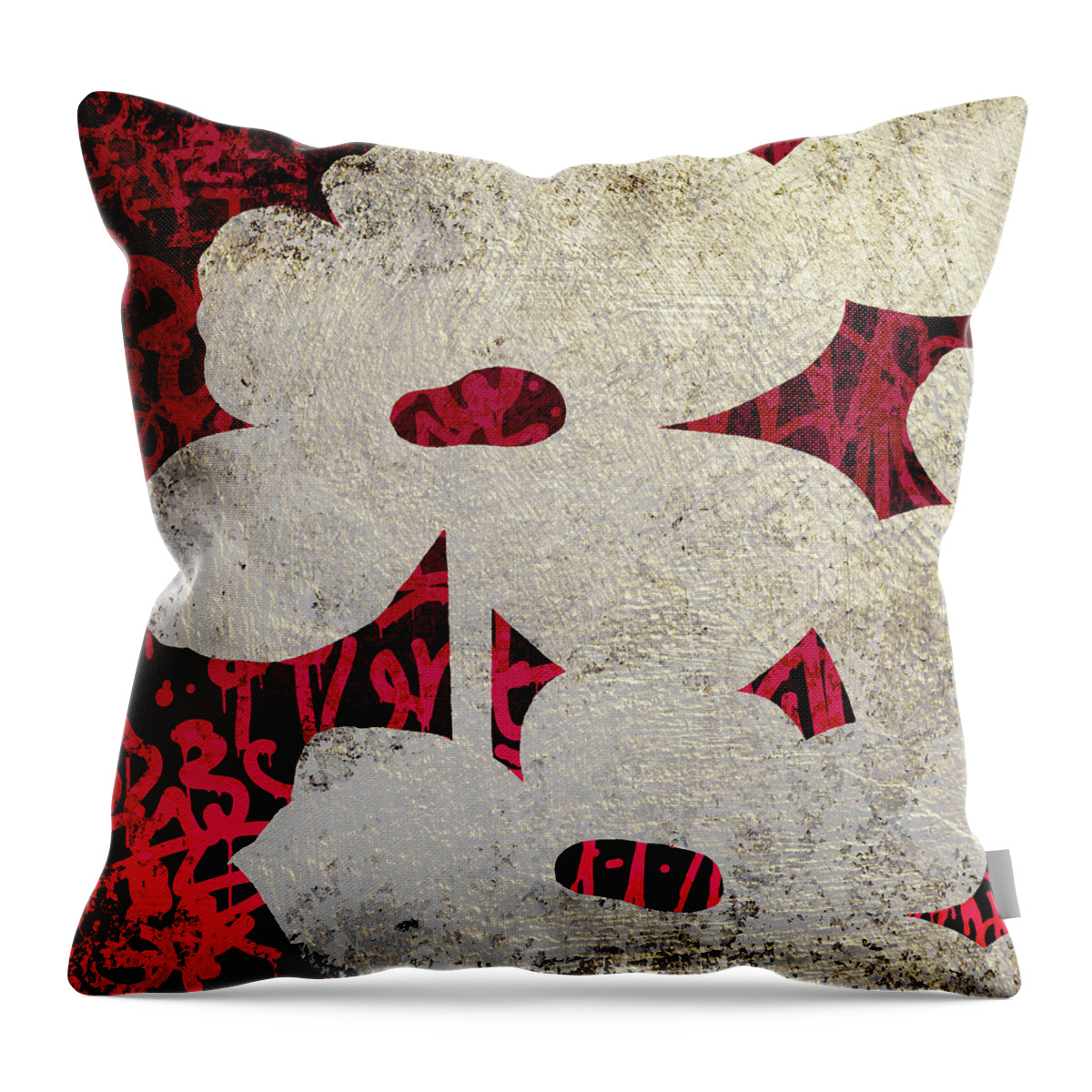This image features a decorative throw pillow that is perfectly square in shape, giving it a soft, puffy, almost cloud-like appearance. The pillow is generously stuffed, causing its corners to point out prominently. Predominantly, the pillow displays a grayish beige color that forms an intricate pattern resembling stenciled outlines of large, oddly-shaped flowers with stems. These flowers are a very light tan, almost white, and cover most of the pillow. However, the gray pattern has several cutouts, revealing a vibrant underlying pattern of dark red and black. This red and black pattern features swirling or squirrely red shapes set against a black background, running prominently along the left side and peeking through various parts of the pillow. Additionally, there is a tag attached to the pillow, possibly indicating its country of manufacture, but the text is not legible from the current angle.